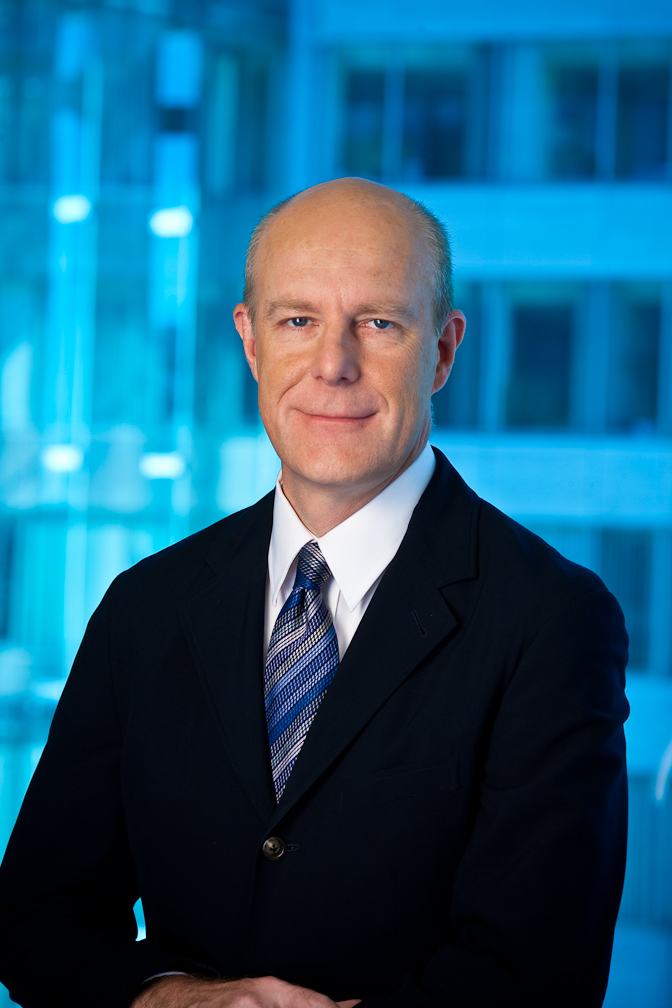In the photograph, a balding man in his mid-fifties, with silver hair at the sides, blue eyes, and a slight smirk, is posing in a seated position. He is dressed in a well-fitted black suit jacket with black buttons, a crisp white shirt, and a tie with diagonal stripes featuring colors such as blue, yellow, purple, and black. His hands rest in front of him on what appears to be a table or his knee. The background reveals a multistory building, possibly an apartment complex, with numerous windows, giving the impression of a cityscape. The building is bathed in a blue hue, which could be a reflection from a window or exterior lighting. The man’s large ears and lack of visible teeth highlight his relaxed yet confident demeanor as he gazes toward the camera.